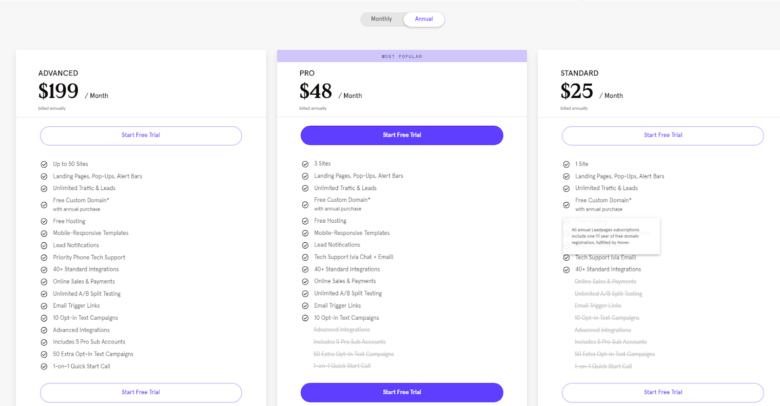A screenshot of a subscription service is displayed, offering users three distinct annual plans for a software platform. The first and most comprehensive option is the "Advanced" plan, priced at $199 per month. This tier includes extensive features such as access to up to 50 sites, customizable landing pages, pop-ups, alerts, unlimited traffic and leads, multiple templates, and lead notifications, making it ideal for high-demand users.

The middle option is the "Pro" plan, available for $48 per month. While not as feature-rich as the advanced tier, it still offers a substantial array of functionalities suitable for moderately demanding needs.

The third and most basic option is the "Standard" plan, which costs $25 per month. This package provides essential features for users with more straightforward requirements.

In this screenshot, the "Pro" package at $48 per month is selected, indicating the user's preference for a balanced mix of features and cost-efficiency.